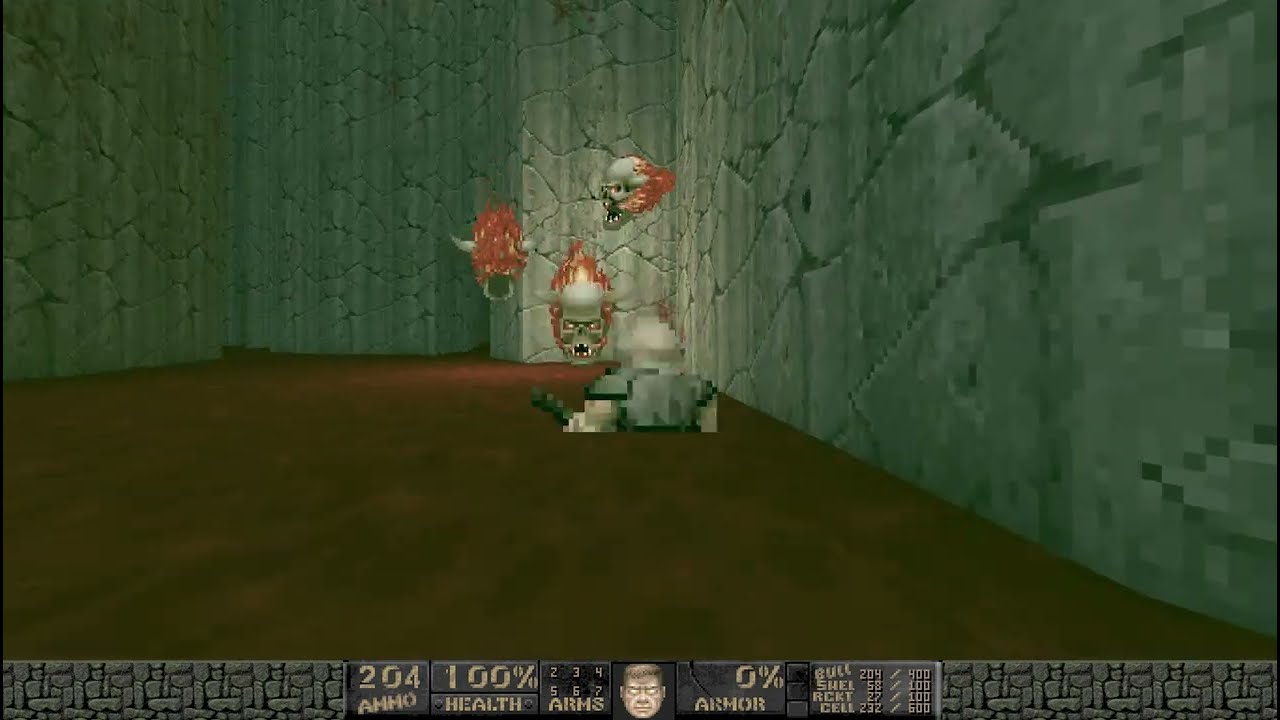The image is a screen capture from an older, possibly pixelated, demonic shooter video game. The scene depicts a room with a white floor and grey, stone walls—one on the far back and another on the right side, forming perpendicular boundaries. Three floating skulls, each with flames emanating from them, occupy the air in front of the walls. The skulls are distinct, with one featuring bull-like horns and the others being human skulls, including one with side horns. Below the floating skulls is a blurry, half-visible human figure, facing away and dressed in grey armor with a brown crown. At the bottom of the screen is a navigation bar with a light brown-on-dark brown text display showing game statistics: 204 ammo, 100% health, ARM 234567, and 0% armor. There is also an image of a man's face with glowing eyes, and details about upgraded weapon costs.